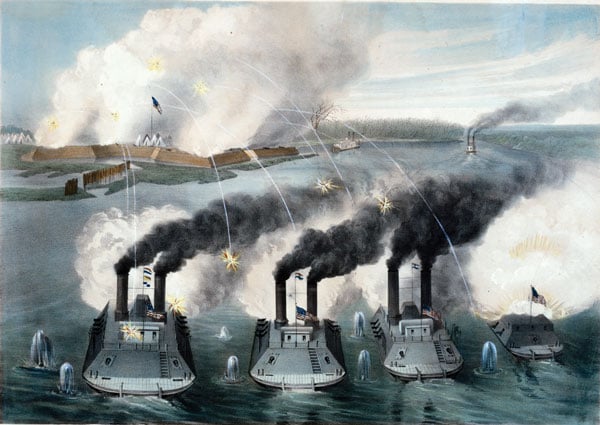The image depicts a chaotic naval battle scene rendered with detailed, grayscale hues, lending it a somber tone. In the foreground, four military boats of varying sizes dominate the composition. The largest boat is on the far left, followed by two medium-sized boats, and finally, a smaller vessel to the far right. Each of the first three boats is equipped with two smokestacks billowing thick black smoke. The smaller boat prominently displays an American flag at its pinnacle. 

Further back, another vessel with similar smokestacks is partially obscured, joined by another indistinct boat in the background. To the left, a fortified structure looms, suggesting a military target under siege. The sky above the fort is alight with what appear to be fireworks, but upon closer inspection, they reveal themselves to be artillery fire or missiles, intensifying the battlefield's chaos. 

The water in the foreground is choppy, adding to the tumultuous atmosphere. Smoke from explosions blends seamlessly into the clouds above, creating an almost apocalyptic skyline. There are small figures, possibly soldiers in white uniforms, discernible near the fort, emphasizing the human element amidst the mechanical warfare. Overall, the image vividly captures the intensity and destruction of a naval battle, with its intricate details painting a stark picture of war.